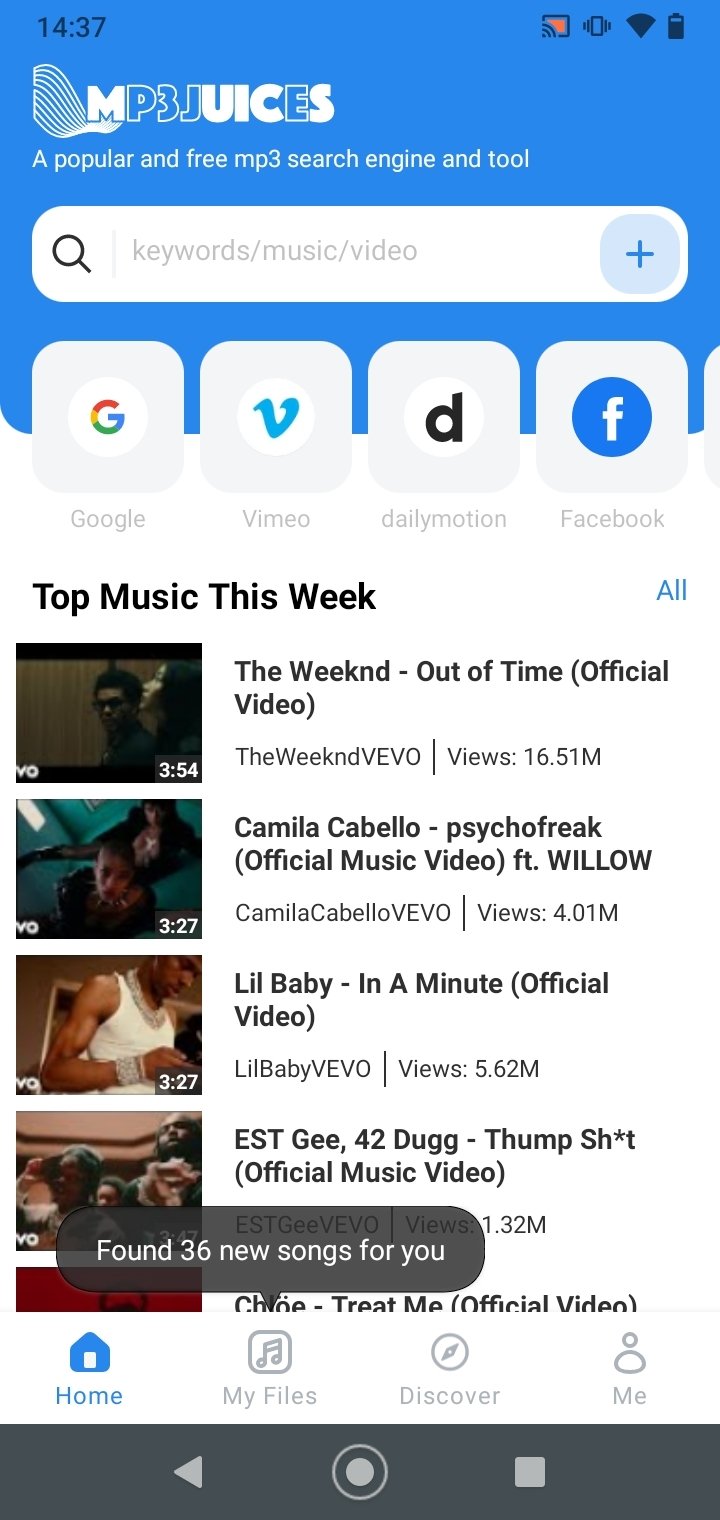Here's a cleaned-up and detailed caption for the described image:

---

This is a screenshot of a phone music application at 14:37. At the top, various icons are displayed from left to right: an orange casting-to-screen logo, a vibrating phone icon, a Wi-Fi signal icon in black, and a battery icon showing approximately 80% charge. Below these icons is the app's logo, "MP3 Juices," a well-known and free MP3 search engine and tool, set against a white background.

Positioned beneath the logo is a white search bar featuring a magnifying glass icon on the left and a plus icon on the right. Directly below the search bar, there are four buttons, each represented by a round logo within a light gray square. These icons are, from left to right: Google, Vimeo, Dailymotion, and Facebook.

In the section below, the heading "Top Music This Week" is displayed in black text, with a blue "All" label to its right. The main content area showcases four music video thumbnails arranged vertically, each with a somewhat darkened thumbnail and a timestamp at the bottom right, except for the last one which is obscured.

1. **The Weekend - "Out of Time" (Official Video)**
   - Uploaded by The Weekend Vivo
   - Views: 16.51 million
   - Duration: 3 minutes 54 seconds

2. **Camila Cabello - "Psycho Freak" (Official Music Video featuring Willow)**
   - Uploaded by Camila Cabello Vivo
   - Views: 4.01 million
   - Duration: 3 minutes 27 seconds

3. **Lil Baby - "In A Minute" (Official Video)**
   - Uploaded by Lil Baby Vivo
   - Views: 5.62 million
   - Duration: 3 minutes 27 seconds

4. **ESTG & 42 Dugg - "Thump Shit" (Official Music Video)**
   - Uploaded by ESTG Vivo
   - Views: 1.32 million
   - Duration: Not visible (obscured)

This structured layout makes it easy for users to search for and explore popular music videos within the application.